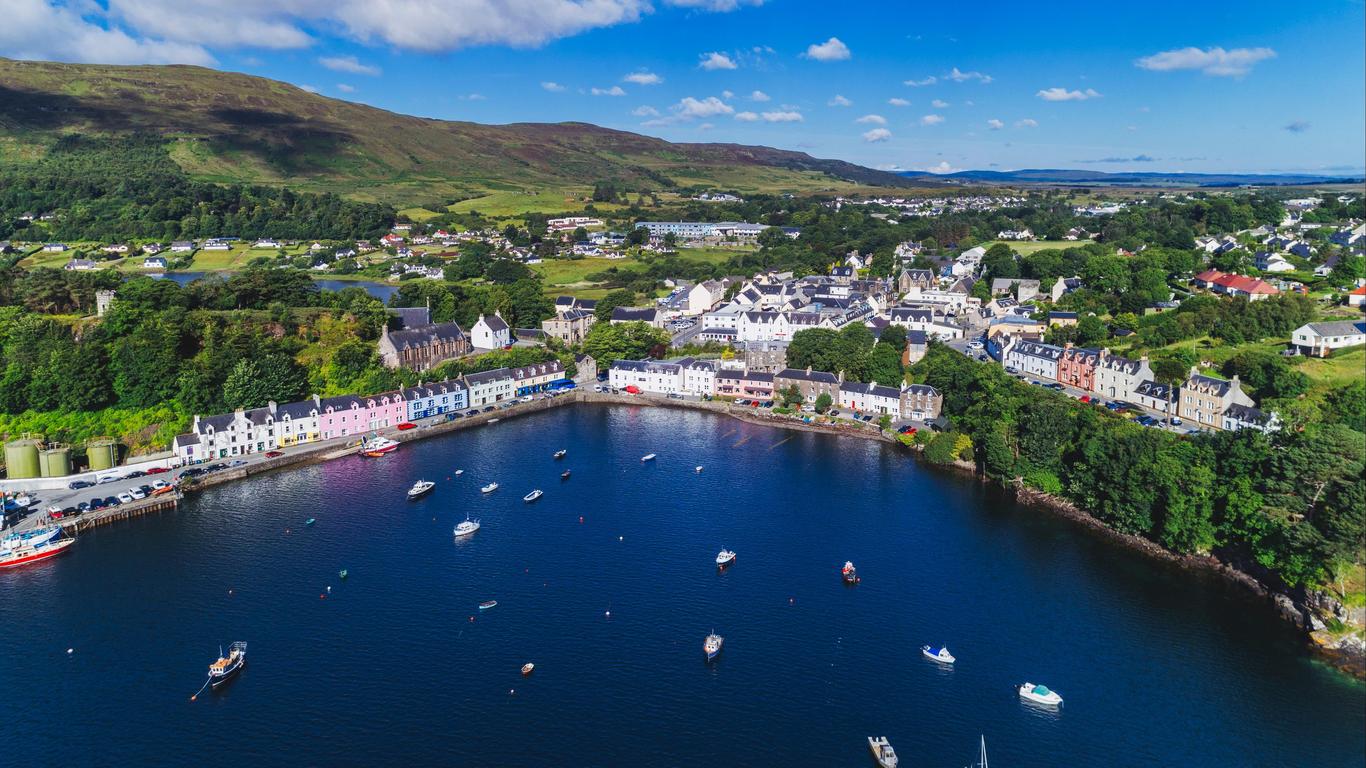This stunning aerial photograph captures a vast, serene lake framed by a picturesque resort area that appears to be nestled within a lush, mountainous landscape. The lake, an intense dark blue, is dotted with numerous small boats, hinting at recreational activities. At the lake's edge, a semicircle of white buildings with red and blue trims, possibly condos or townhouses, create a charming waterfront scene reminiscent of Scandinavian architectural styles. Beyond these buildings, the landscape transitions into verdant greenery and rolling hills, with a mix of taller lush trees and cozy neighborhoods visible throughout the expanse. The right side of the lake is undeveloped, offering a stark contrast with its dense tree coverage. In the distance, majestic mountains rise gradually, providing a backdrop to this scenic area. Additionally, there is a hint of another smaller body of water to the left of the main lake. The vibrant blue sky overhead is adorned with patches of white clouds, accentuating the natural beauty of this tranquil resort setting.